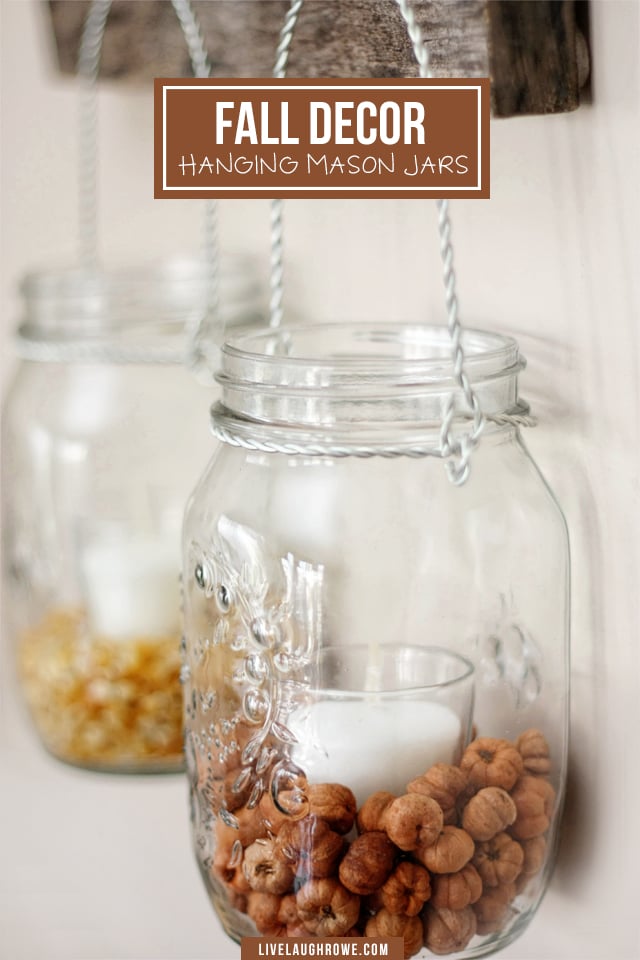This image is a modern DIY-style advertisement for "Fall Decor Hanging Mason Jars," featuring a rustic, autumnal theme. The display includes two clear mason jars hanging from a wooden beam, each with wire wrapped around the top to create a hanger. The jars are filled with various decorative items such as acorns, popcorn, or possibly nuts and small baby pumpkins. Inside one of the jars is a votive candle, cleverly designed to resemble a shot glass of milk. The jars are positioned against a wooden backdrop, with an advertisement sign at the top that reads, "Fall Decor Hanging Mason Jars." A website link, LiveLifeRowe.com, is displayed at the bottom, suggesting this is likely an online ad one might find on Pinterest or Etsy.